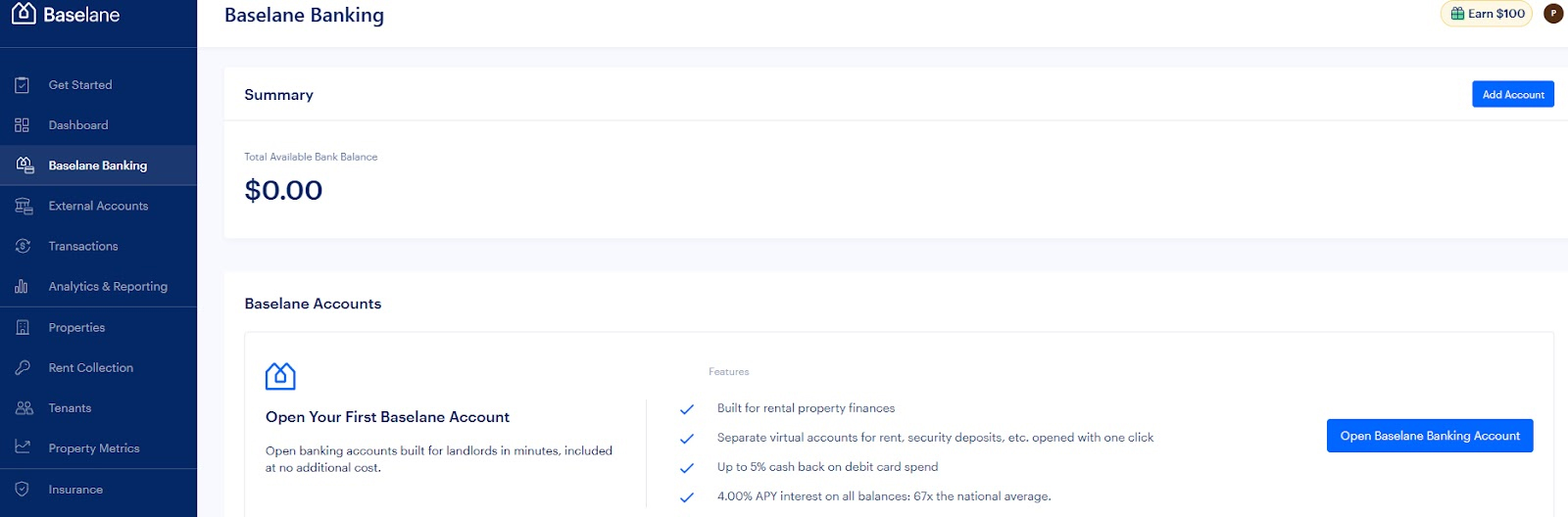The landing page for Baselane, an online bank designed for landlords, prominently features the Baselane Banking section. At the top, the page displays "Baselane Banking" in blue, followed by a "Summary" header. On the far right, there is a blue "Add Account" button. Directly below, a section titled "Total" displays "Total Available Bank Balance" in small, light gray text, alongside a balance of $0.00.

The page further details Baselane's offerings. Under "Baselane Accounts," users are encouraged to "Open Your First Baselane Account." This is followed by a description stating, "Open Banking Accounts Built for Landlords in Minutes Included at No Additional Cost." To the right, a feature list highlights advantages such as:

- Built for Rental Property Finances (check mark)
- Separate Virtual Accounts for Rent, Security Deposits, etc., Opened with One Click (check mark)
- Up to 5% Cash Back on Debit Card Spend (blue check mark)
- 4% APY Interest on All Balances, 67 Times the National Average

Adjacent to these features, a prominent blue button with white text invites users to "Open Baselane Banking Account."

On the far left, a vertical blue menu lists several navigational options in white text, starting with "Baselane" at the top, followed by:

- Get Started
- Dashboard
- Baselane Banking (highlighted as the current selection)
- External Accounts
- Transactions
- Analytics and Reporting
- Properties
- Rent Collection
- Tenants
- Property Metrics
- Insurance